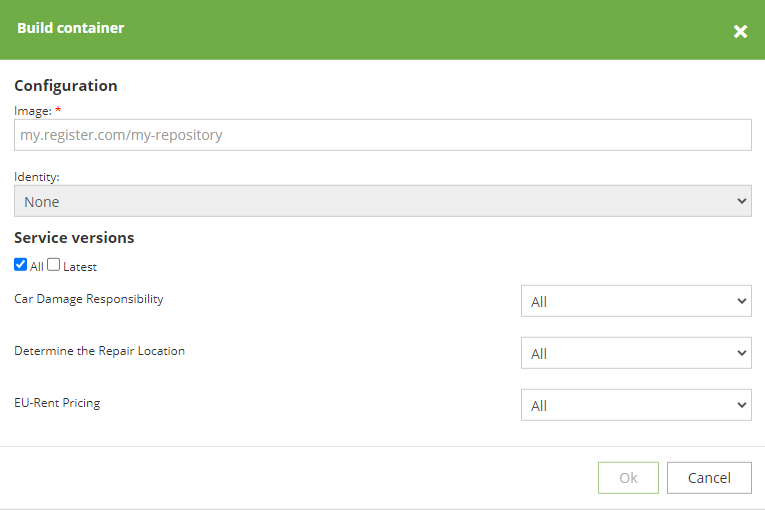This image depicts a user interface with a predominantly white background, except for a dark green border about an inch thick along the top. In the top-left corner, there is a bold, white container with the word "Build" and on the top-right, a bold white "X." Below this, the background remains white. 

On the left side of the interface, the bold black text reads "Configuration," followed by the label "Image" in regular black text marked with a red asterisk. Directly below, a large white rectangular field spans across, bordered in gray, containing the URL "my.register.com/my-repository" in gray text.

Underneath the image section, the black text label "Identity" is followed by a gray rectangle that extends across the interface with the word "None" inside. Below this, the bold text "Service Versions" is followed by a section featuring a blue square with a white checkmark to its left, labeled "All" in black text. Adjacent to this, a white square with a black border is labeled "Latest." Further below, the text reads "Karma Damage Responsibility" in black.

On the right side of the interface, there's a dropdown tab with a white and gray border that has the word "All" in black. Moving to the left, the following section reads "Determine the Repair Location," with another similar dropdown tab containing the word "All." Below that, in the left section, it says "EU Rent Pricing," which is again paired with a dropdown tab labeled "All." At the bottom, a small section with a gray border is visible.

In the bottom-left corner of the interface, there is a white button with a black border labeled "Cancel." To its right, another white button with a gray border displays the text "Okay" in gray. Beneath these buttons is an additional horizontal element with a gray border.